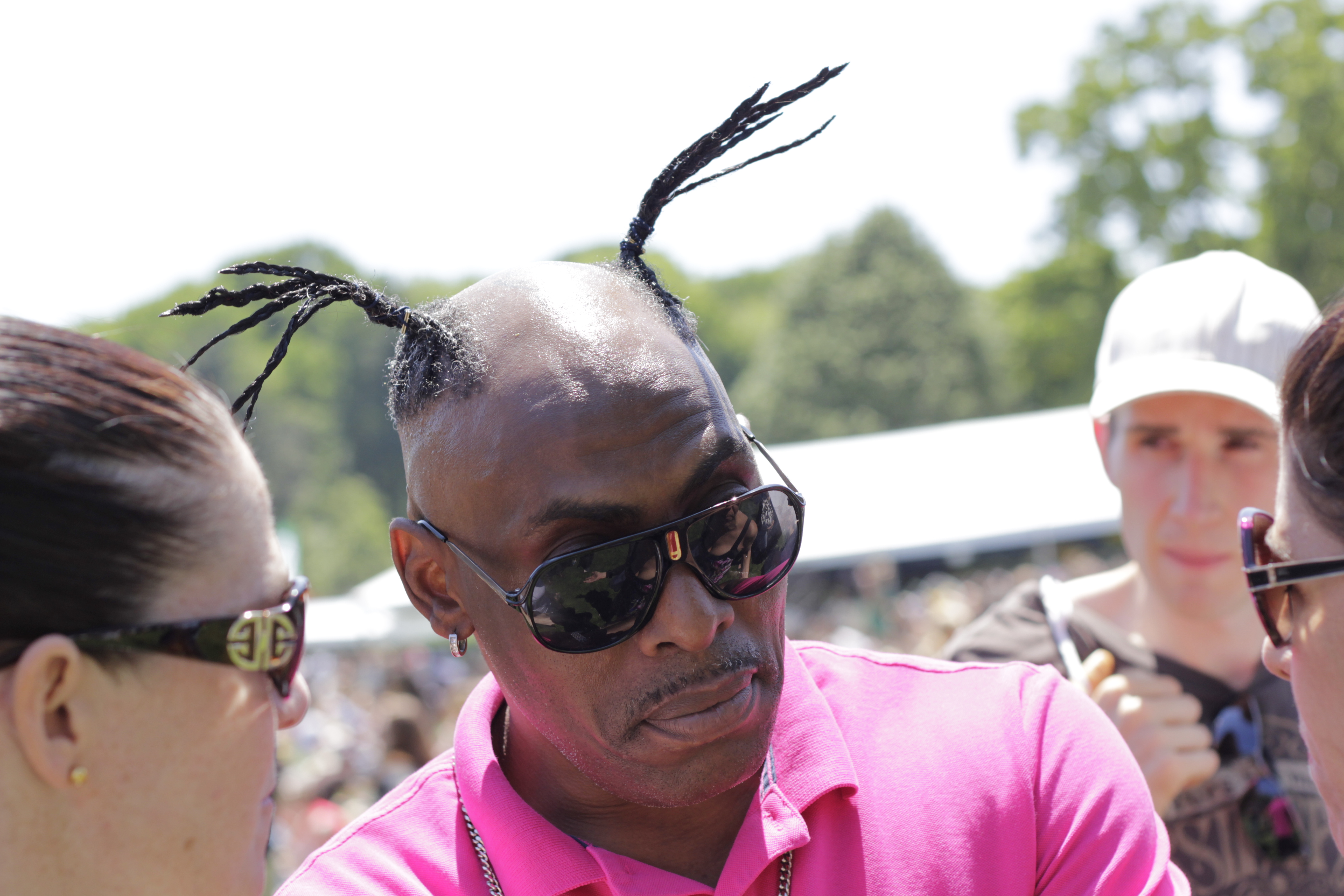In the image, we observe a busy outdoor setting. The top portion of the image showcases a bright sky flanked by a canopy of trees. Below this, a bustling crowd of people is visible, along with several buildings and structures that form the backdrop. Dominating the center of the image is a man wearing sunglasses and sporting a quirky hairstyle, facing towards the right. The photograph is devoid of any textual elements. The color palette includes shades of white, green, brown, black, tan, gold, and pink, contributing to the vibrant scene. The setting appears to be a park, captured in the middle of the day, likely during a lively event.